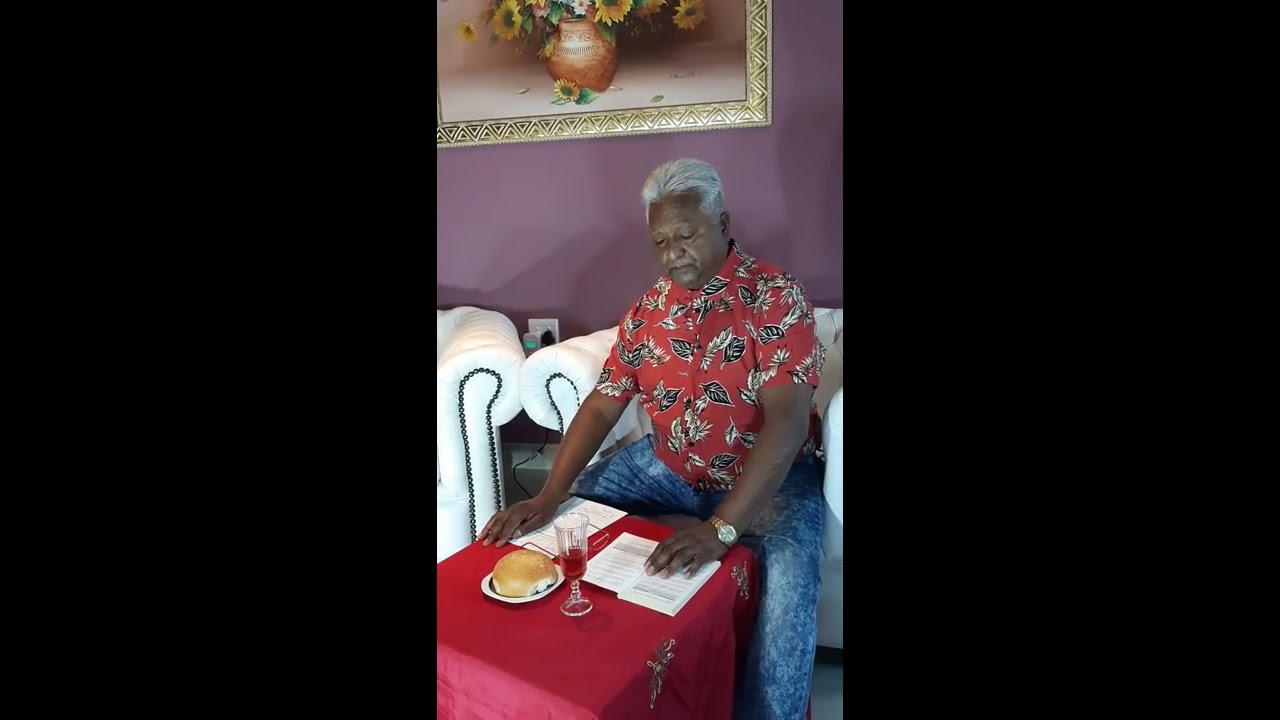In this detailed indoor photograph, an older Indian man with graying short hair and dark skin is seated on a plush, white single-seater sofa adorned with black beading. His expression is calm, eyes downcast or perhaps closed, as he focuses on some papers or an open book lying on a small, square table draped in a red tablecloth in front of him. He is wearing a Hawaiian-style red shirt featuring black and white leaf patterns paired with blue jeans. The man sports a gold watch on his wrist. On the table, there's a round bakery bun on a plate, a pair of eyeglasses, and a crystal goblet filled with a deep red liquid, possibly wine or juice. The room has purple walls, and a partially visible painting of a flower pot filled with vibrant flowers hangs behind him. Vertical black strips frame the sides of the image, adding a structured contrast to the scene.